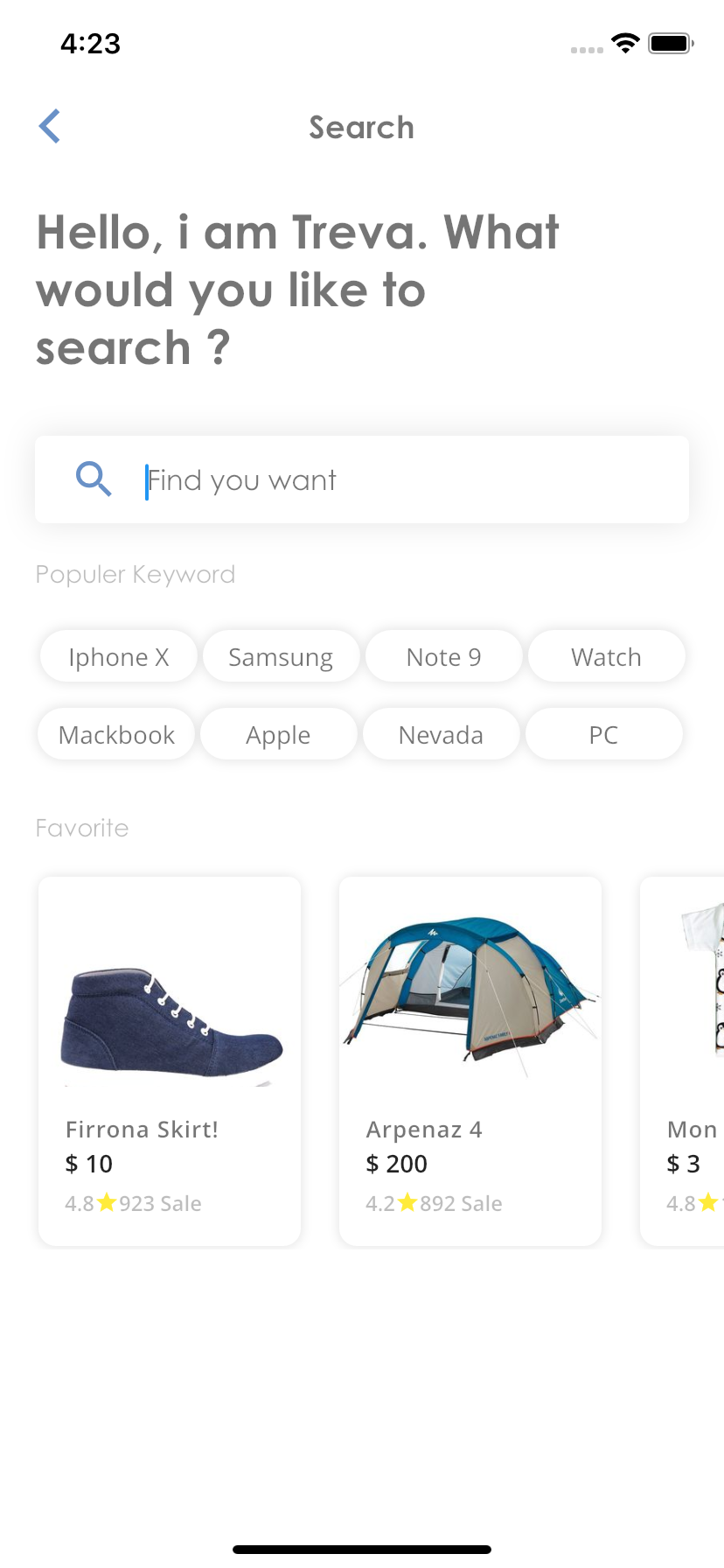The screenshot, taken from a cell phone, showcases a product information page, likely for various gear items. At the bottom of the image, three sections display different products and their details, listed from left to right. 

The first section features a purplish shoe pointing to the right. The text underneath reads "FIRRONA skirt for $10" with a rating of 4.8 stars and "923 sales."

The second section displays an image of a tent, with the text "ARPENAZ for $200" below it. This product has a rating of 4.2 stars and "892 sales."

The third section is partially cut off, showing only the letters "MON" and a dollar sign followed by the number three. This product also has a rating of 4.8 stars, indicated at the bottom of the image.